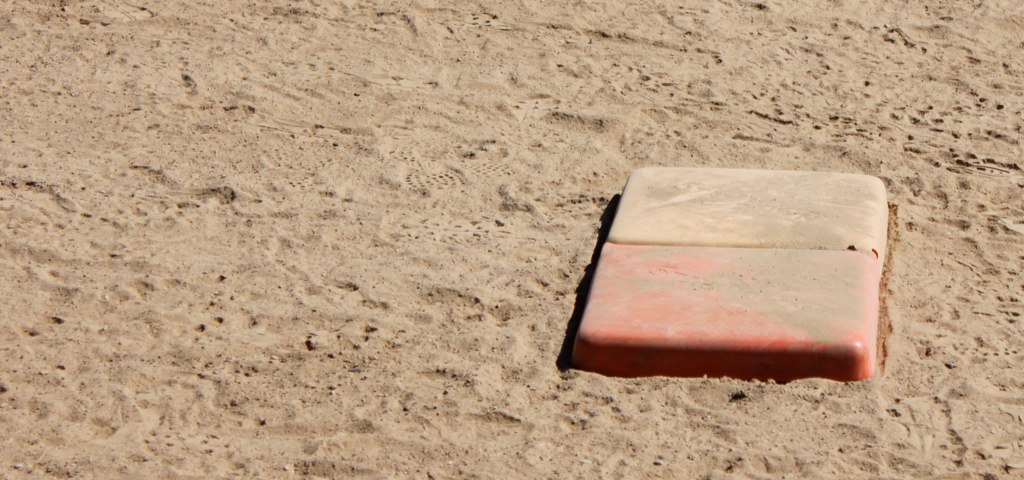The photograph depicts a section of a baseball field on a sunny day, focusing on a base that appears to be either under development or distinctly different from typical baseball bases. The base is orange at the bottom and white or yellow at the top, featuring a noticeable horizontal line that divides it in half. The top section is smeared with dirt. Surrounding the base, the ground consists of clay-like dirt with numerous cleat marks indicating recent activity. The image is rectangular in shape, capturing the base casting a prominent shadow, adding depth and contrast to the scene. The overall texture of the dirt is similar to windblown sand, showing small pits and grooves. Additionally, there seems to be another white rectangular object adjacent to the orange base, which may serve the purpose of reducing collisions, possibly indicating a placement for safety during games, commonly seen in youth or high school leagues.